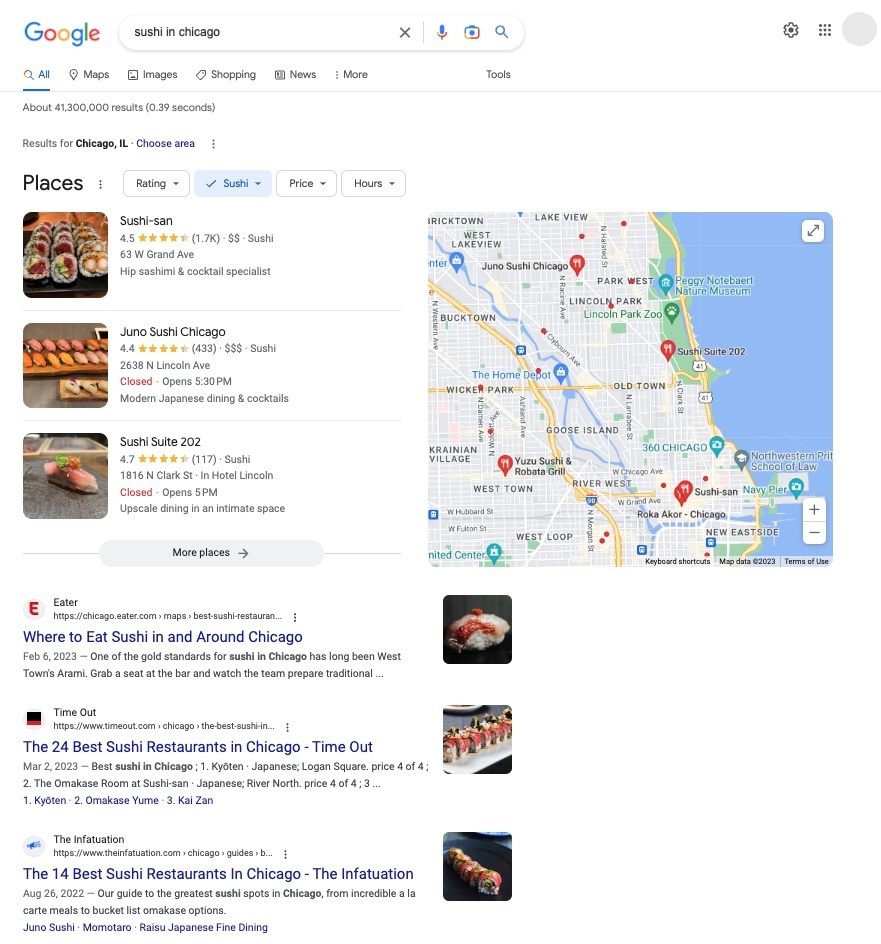This is a detailed screenshot of Google search results for "sushi in Chicago." In the top left corner, the familiar Google logo is displayed next to the search bar containing the user's query. Directly below the search bar are various tabs associated with the search, with the "All" tab currently highlighted in blue and underlined. Adjacent tabs include "Maps," "Images," "Shopping," "News," and a "More" dropdown, along with a "Tools" button.

The results section reveals that the search yielded approximately 41,300,000 results. The first result is "Sushi-san," boasting a 4.5 out of 5-star rating based on 1.7 thousand reviews. This mid-range restaurant is described as a "hip sashimi and cocktail specialist." 

Next is "Juno Sushi Chicago," which holds a 4.4 out of 5-star rating with 433 reviews. It is noted for being a pricey option and is currently closed, reopening at 5:30 p.m. This establishment offers "modern Japanese dining and cocktails."

The final result is "Sushi Suite 305." The entry details for this establishment are truncated in the screenshot and not entirely visible.